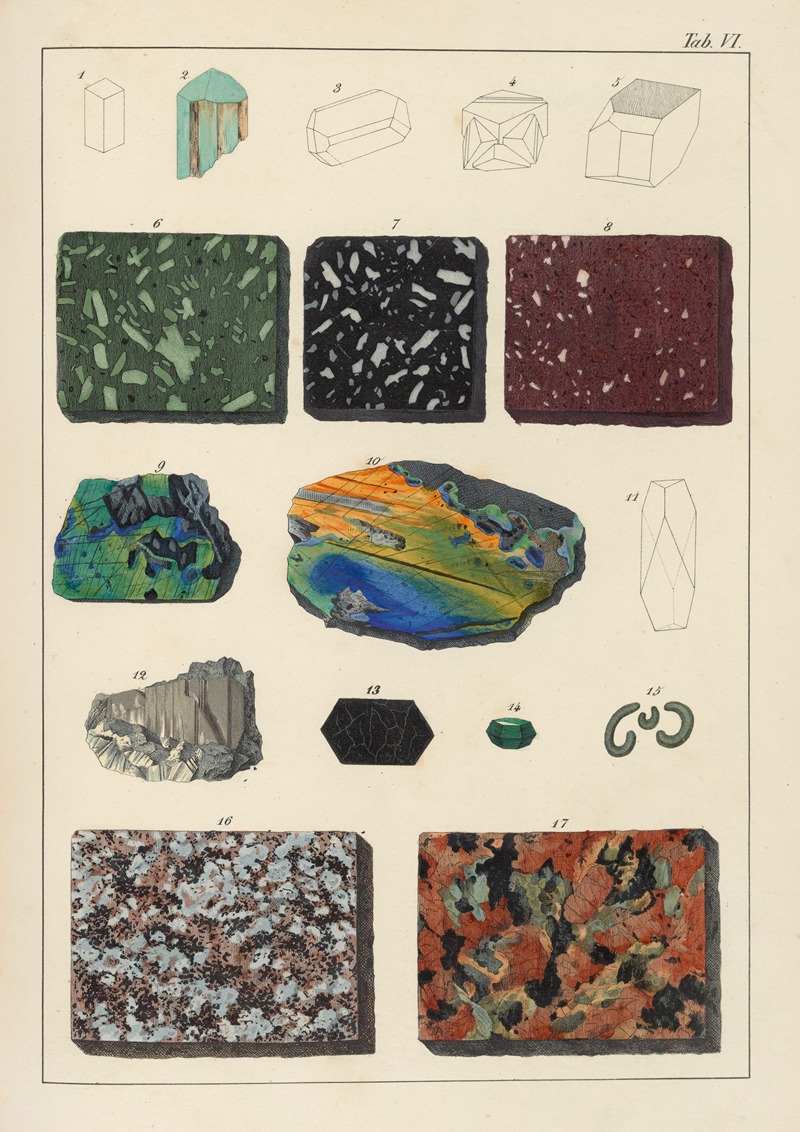In this image, a collection of 17 different types of rocks and mineral samples is meticulously arranged and numbered from 1 to 17. At the top right corner, there's a small inscription, "tab 17," in black font. The rocks are displayed in several rows, each with distinct characteristics:

- The first row (topmost) includes rocks numbered 1 through 5. Most of these are structural illustrations, with the exception of number 2, which is turquoise-colored.
- The second row features numbers 6, 7, and 8. These are slab-like and colorful, resembling polished countertops. Number 6 is green, number 7 is black and white, and number 8 is a dark purplish-red.
- The third row shows numbers 9, 10, and 11, which look like portions of rock surfaces. Numbers 9 and 10 exhibit intricate patterns with blue, turquoise, green, yellow, and black hues, while number 11 is just an outline without any color.
- The fourth row, containing numbers 12, 13, 14, and 15, showcases additional mineral samples. Number 12 is gray and looks like a mineral, number 13 is small and black, number 14 is emerald-green and the smallest image, and number 15 appears as a couple of gray hooks.
- The final row at the bottom consists of two larger, square tiles, numbered 16 and 17. Number 16 resembles a granite countertop with a mix of white, black, and light purple, while number 17 is salmon-colored with hints of yellow and black.

This detailed arrangement highlights the diverse textures, colors, and patterns of the rocks and mineral samples, from structural drawings to vividly polished slabs.